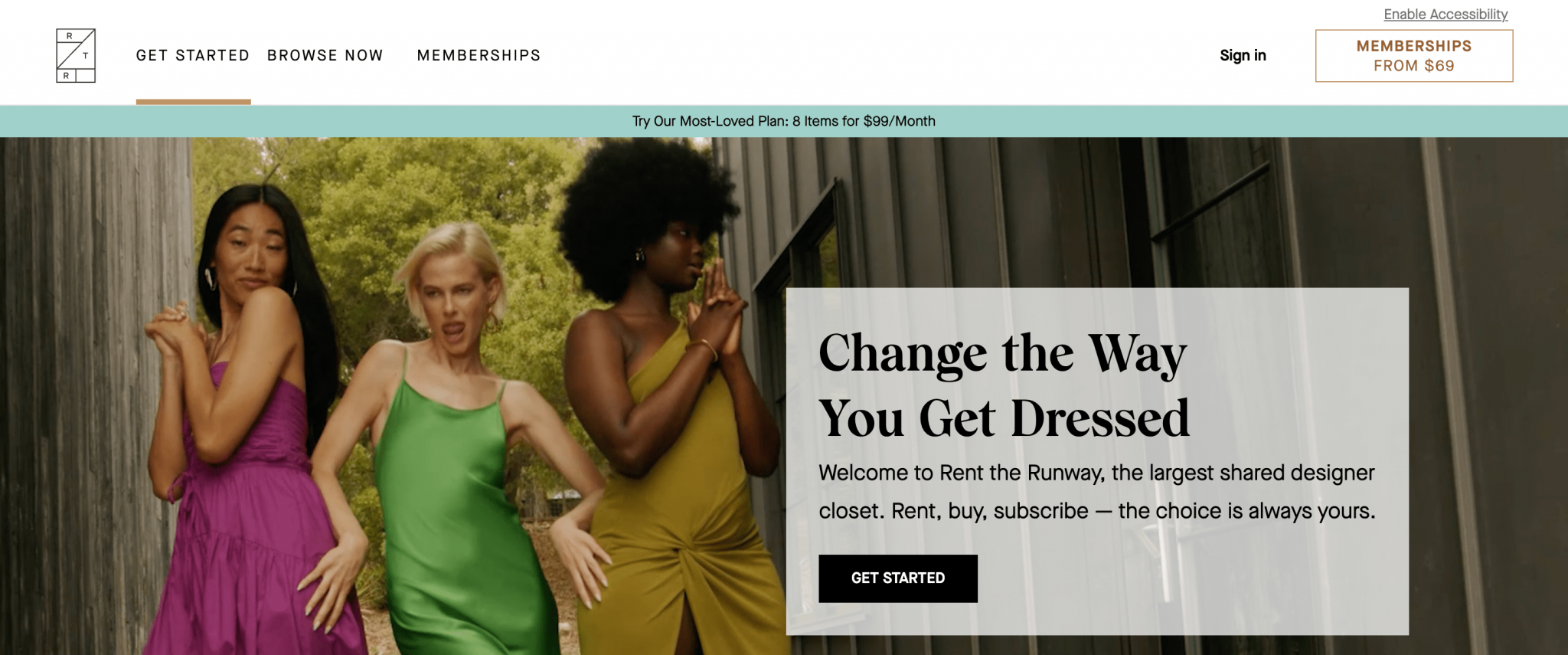This detailed image showcases a fashion website interface. 

Key features include:
- **Header**: In the upper left corner, there's a distinctive rectangular logo box featuring letters and triangular shapes.
- **Navigation Bar**: 
  - Left to right: "Get Started" (underscored), "Browse Now," and "Memberships."
  - Right side: "Sign In," and a rectangular box highlighting "Memberships from $69."
- **Above Membership Section**: An underscored link labeled "Enable Assembly."
- **Banner**: 
  - Just below the membership section, there's an eye-catching aqua green banner with the text "Try Our Most Loved Plan."
  - The banner offers an enticing message, "8 Items for $99 a Month."
- **Main Content**:
  - A large, central media image features three women striking unique poses, wearing vibrant dresses: one in purple, one in green, and another in gold.
  - Accompanied by the slogan, "Change The Way You Get Dressed," set against a faded gray background.
  - Below, the welcoming message reads, "Welcome to Rent the Runway, the largest shared designer closet. Rent by subscription - The choice is always yours."
  - The section concludes with a prominent "Get Started" button housed in a black rectangular box.

The overall design succinctly conveys the website's offerings and facilitates easy navigation for users.